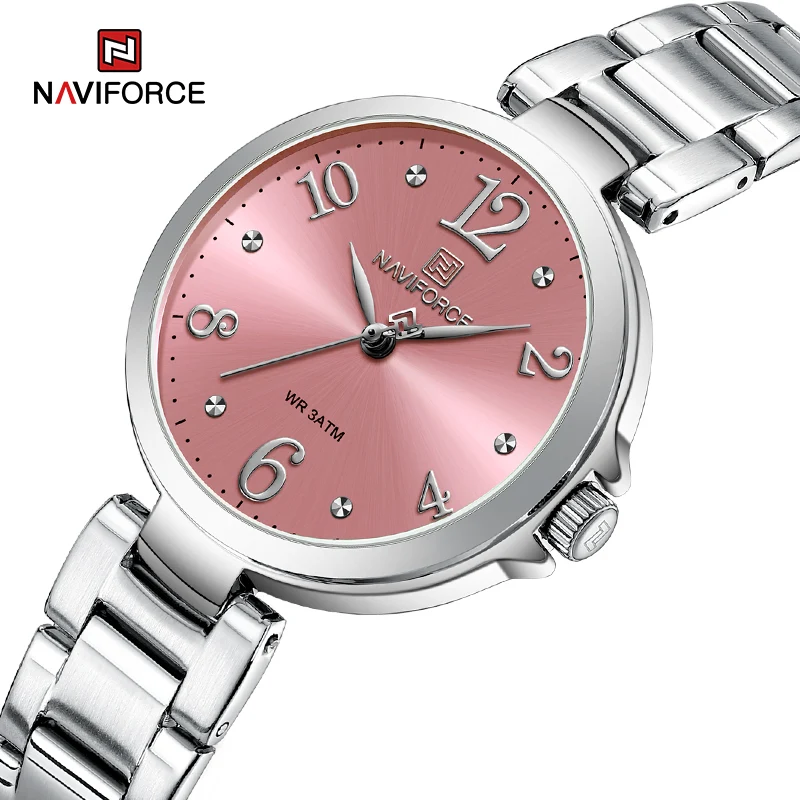This close-up image prominently features a stylish Naviforce watch set against a white background. The watch boasts a slender linked silver band that extends towards the upper right and lower left of the frame. The medium-sized dial face, bathed in a pink or rose hue, showcases a harmonious blend of silver elements. The 12, 2, 4, 6, 8, and 10 markers are in silver, interspersed with diamond-like stones representing the odd numbers. The silver hour, minute, and second hands complement the overall aesthetic. In the upper left corner, the distinctive Naviforce logo— a red square with intertwined white arrows forming an 'N'— is clearly visible, accompanied by the brand name NAVIFORCE in black, with a red 'A'. The face is further detailed with the inscription “WR3ATM” just above the 6 o'clock position. Overall, this image exudes the refined elegance of the timepiece, perfect for use in a shopping graphic or detailed product description.